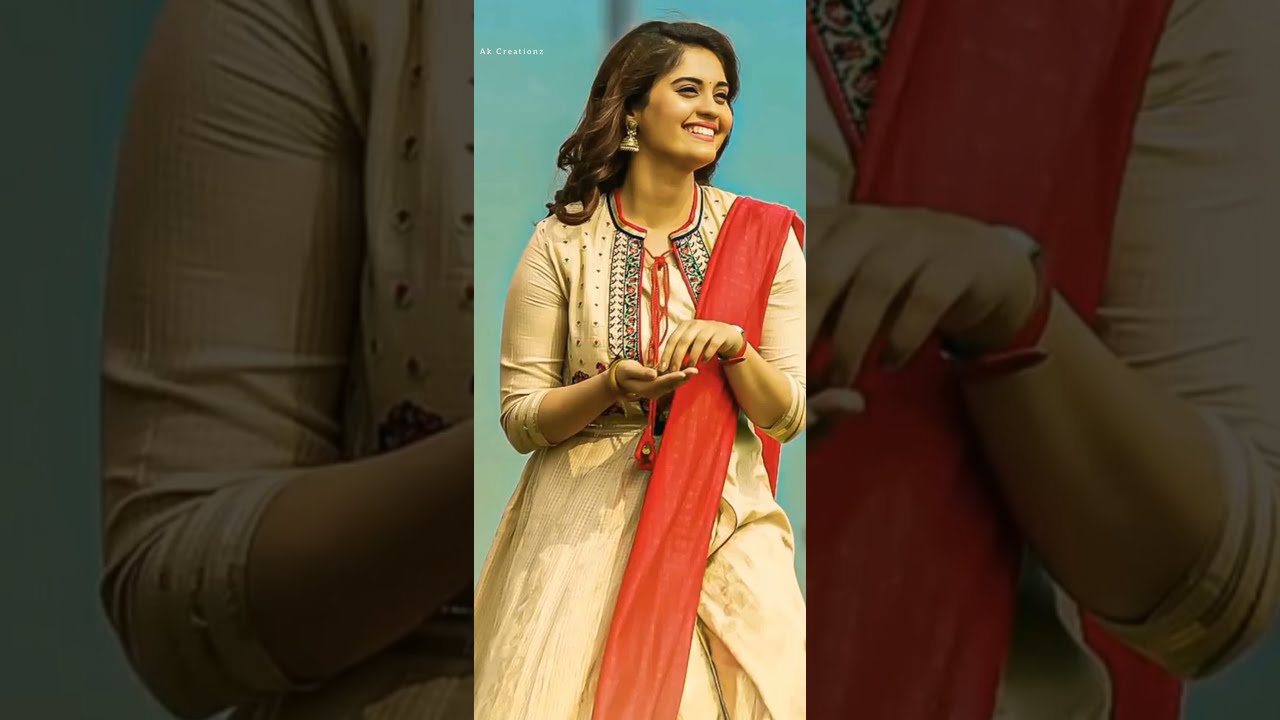The image is a detailed portrait of a young woman, likely of Indian descent, with medium skin and shoulder-length dark brown hair that flows to her right. She is smiling warmly, revealing the top row of her teeth, and her eyes are nearly closed. She wears a cream-colored dress with intricate designs, including decorative panels running down the front. The dress covers her arms up to just past the elbows, while her forearms are exposed. Around her neck is a collar featuring red, white, and blue, and it is tied at the center with a red ribbon. Vertical floral designs add to the elegance of the dress, which also extends out of the frame, hinting at its length beyond her knees. Draped over her left shoulder is a long red scarf (dupatta), which flows behind her.

The woman is accessorized with a gold bell-like earring in her right ear and a traditional bindi on her forehead. She has her hands in front of her body; her right hand is holding an object that she is touching with her left pointer finger.

The photograph itself is centered within a landscape-oriented frame measuring approximately six inches wide by three inches high. To fill the space around the central vertical image, the sides feature darkened and enlarged close-ups of her right and left arms and the upper part of her dress. The background is predominantly blue, providing a contrasting backdrop to her attire.